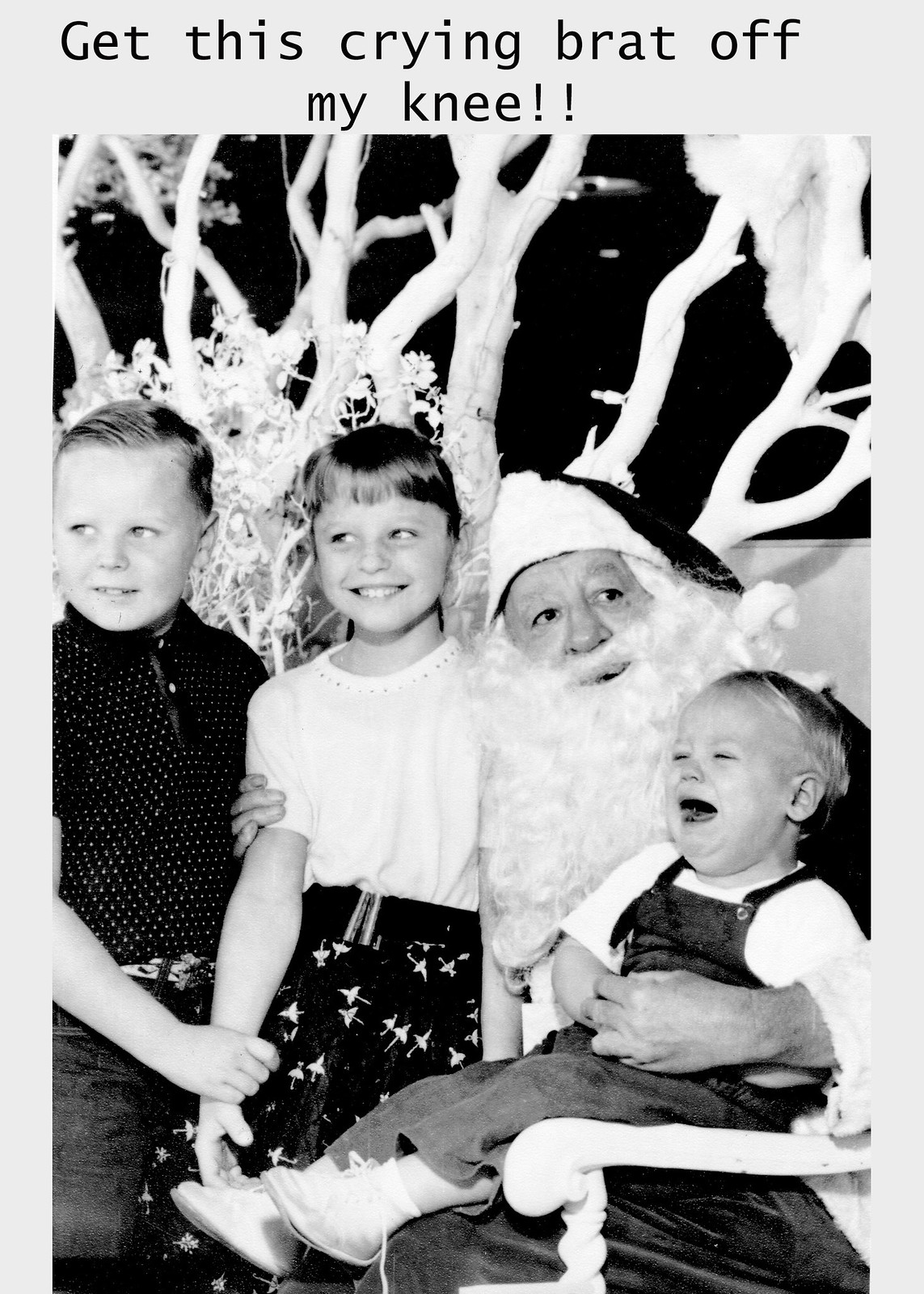This black-and-white photograph, formatted like a Christmas greeting card and set against a white mat, captures a humorous holiday scene with Santa Claus and three children. Santa, seated in a white chair, is surrounded by a festive white tree and a dark backdrop. The title above the image humorously reads, "Get This Crying Brat Off My Knee!!". 

In the center, a small child around two years old sits on Santa's knee, wailing in distress. The child is dressed in overalls, a white t-shirt, and white shoes. Despite the child's tears, Santa appears more resigned than upset, glancing off to the side as if seeking help from the parents. 

Standing to Santa's left are two older children, a girl and a boy, both about six or seven years old, dressed in nice outfits – the girl in a white blouse and skirt, the boy in a collared shirt and jeans with a belt. The girl stands closest to Santa, smiling brightly, while the boy, also smiling, holds her wrist. The contrast between the cheerful older children and the crying toddler, along with Santa's perplexed expression, makes for a comical and heartwarming snapshot of a classic holiday moment.